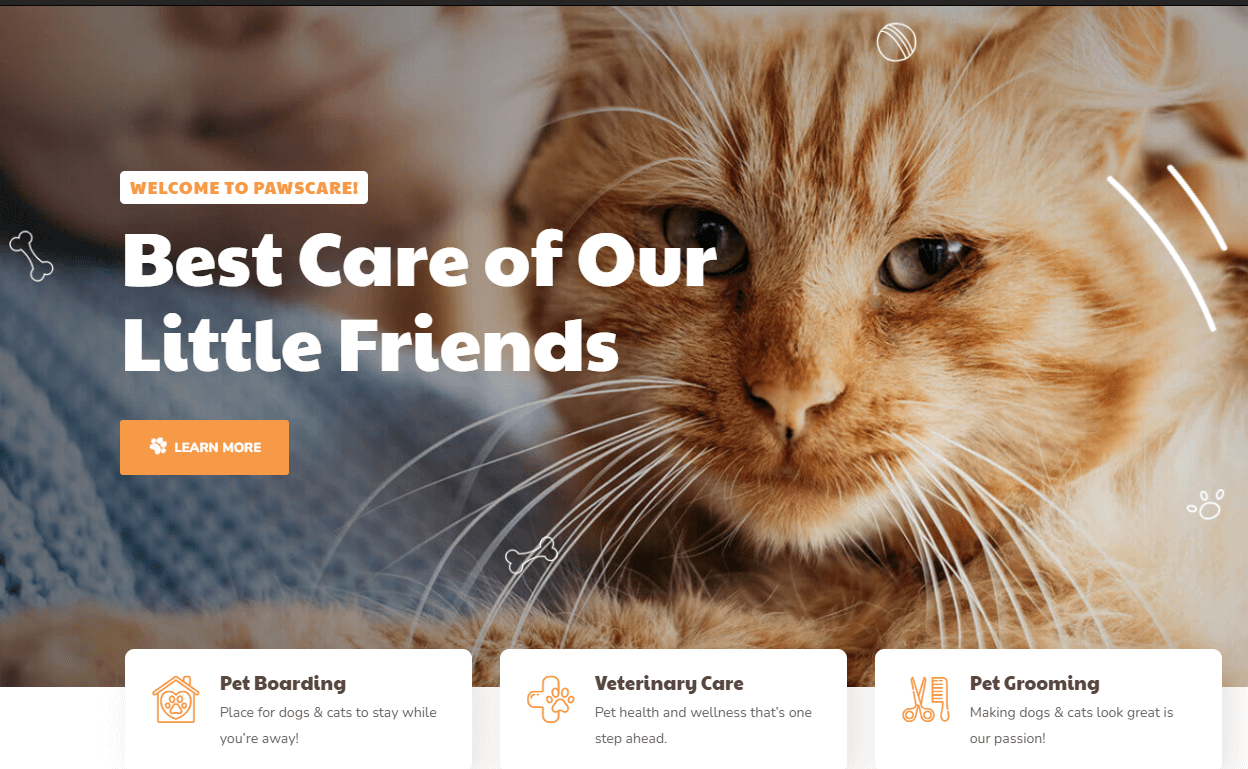The image showcases a clean and visually appealing website with a horizontal layout, approximately one and a half to two times wider than it is tall. Prominently featured in the background is a detailed close-up of the head of an orange cat with striking gray eyes, gazing directly at the viewer. A slightly blurred image of a smiling woman in a blue shirt appears in the upper left corner, adding a personal touch.

Overlaying the background, an inviting banner displays the text "Welcome to Paws Care" in orange letters on a white background, positioned about a third of the way down on the left side. Below, in bold white letters, the slogan "Best Care of Our Little Friends" stands out, with an orange button labeled "Learn More" just beneath it.

The lower section of the website preview features the tops of three horizontally aligned boxes, each dedicated to a different service. "Pet Boarding" highlights a safe haven for dogs and cats while their owners are away, marked with an orange icon of a pet house. "Veterinary Care" emphasizes pet health and wellness with the tagline "One Step Ahead," accompanied by an orange icon of a stethoscope. Lastly, "Pet Grooming" emphasizes their passion for making pets look great, symbolized by an orange icon of grooming scissors.